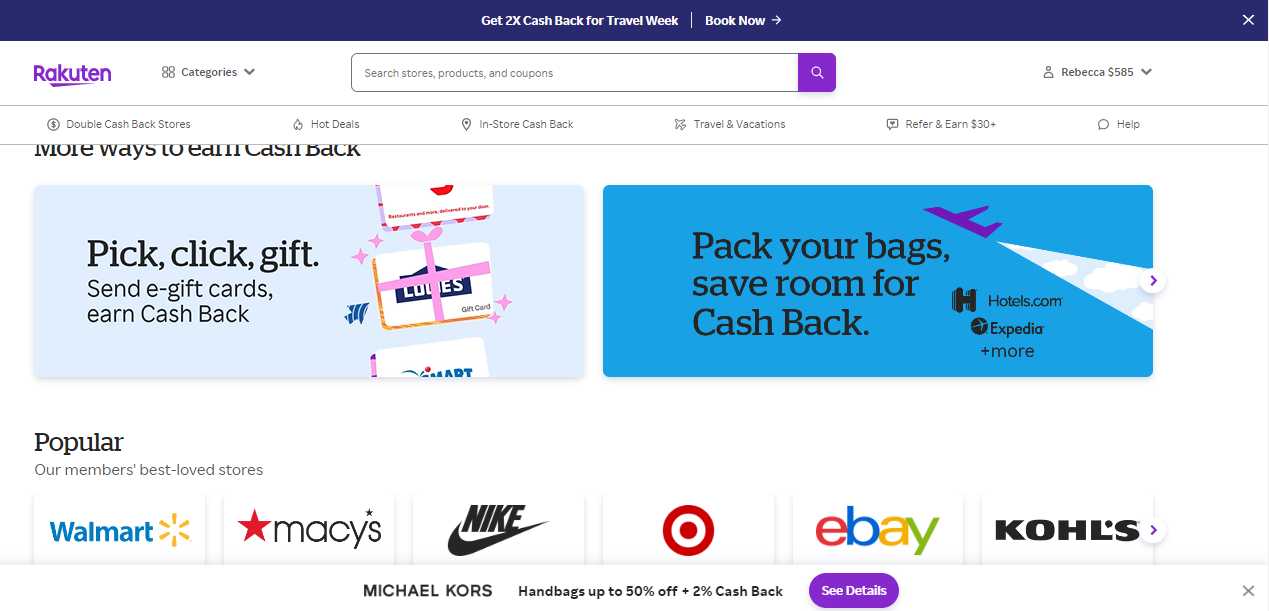This is a screenshot of a web page from the Rakuten website, displaying various shopping options and special deals from different retailers. The top section prominently highlights a special Travel Week promotion offering double cashback rewards. Below this, there appears to be an option to book travel arrangements, likely flights.

The webpage belongs to a user named Rebecca, who is looking to redeem her accumulated rewards or points across several online stores. The retailers listed include Walmart, Macy's, Nike, Target, eBay, and Kohl's. Additionally, there is a highlighted advertisement at the bottom of the page for Michael Kors handbags, showcasing a 50% off sale combined with a 2% cashback offer on any bag purchased. Users can click to see more details about this deal.

Other features on the page include various opportunities to earn double cashback on select purchases, deals for in-store shopping, and an option to refer friends for additional earnings. There is also a customer service help button for users needing assistance.